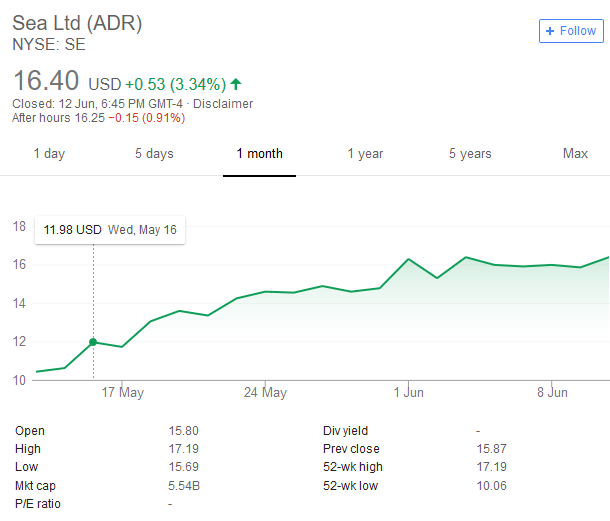The image displays a detailed graph illustrating the fluctuating stock prices of CSEA Limited (ADR) on the New York Stock Exchange Southeast. The graph prominently features a line chart that tracks the stock's progress over specific time intervals: 1 month, 1 year, 5 years, and maximum. On the left side of the graph, the price scale ranges from $10 to $18 USD. Time markers are indicated for May 17th, May 24th, June 1st, and June 8th.

Highlighted at the upper right corner, there is an option to follow the stock. The stock is valued at $1640 USD, marking an increase of 0.53 points or 3.34%, as indicated by the green upward arrow. Additional information specifies that the closing price on June 12th was recorded at 6:45 PM GMT-4. The disclaimer notes an after-hours change of -0.15 points or -0.91%, resulting in a value of 16.25.

The chart shows a notable upward trend, starting at a lower value and rising to its peak, representing the highest value recorded within the displayed timeframe.